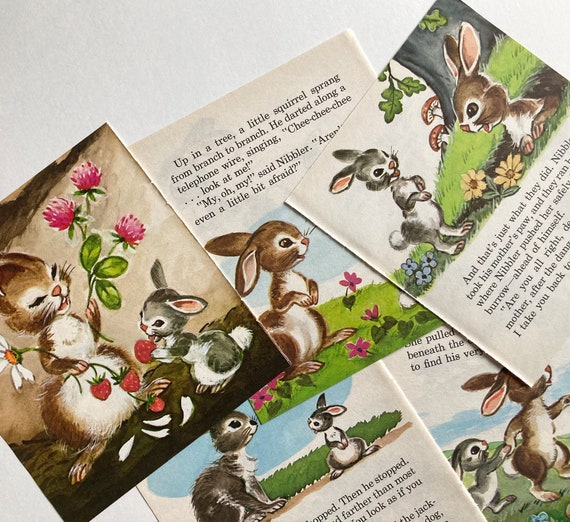The image displays several pages from a vintage children's storybook, possibly dating from the 1960s or early 1970s. The story features adorable bunny characters, notably a mother bunny and her baby bunny, who are depicted holding strawberries and flowers. The charming illustrations, seemingly created with colored pencils, use a pleasant palette of browns, grays, warm greens, and pinks in the flowers, giving the scenes a wholesome, nostalgic feel. The overlapping pages reveal snippets of text narrating a sweet, innocent story, including a scene where Nibbler, the baby bunny, interacts with a squirrel and another where Nibbler and his mother run together hand-in-paw. Although the text is partially obscured, it suggests a tale full of gentle adventures and curiosity. The arrangement of the pages suggests they might have been torn out and layered for display, evoking the timeless appeal of classic children's literature, which could easily be found in antique stores or thrift shops, still enjoyable for children today.